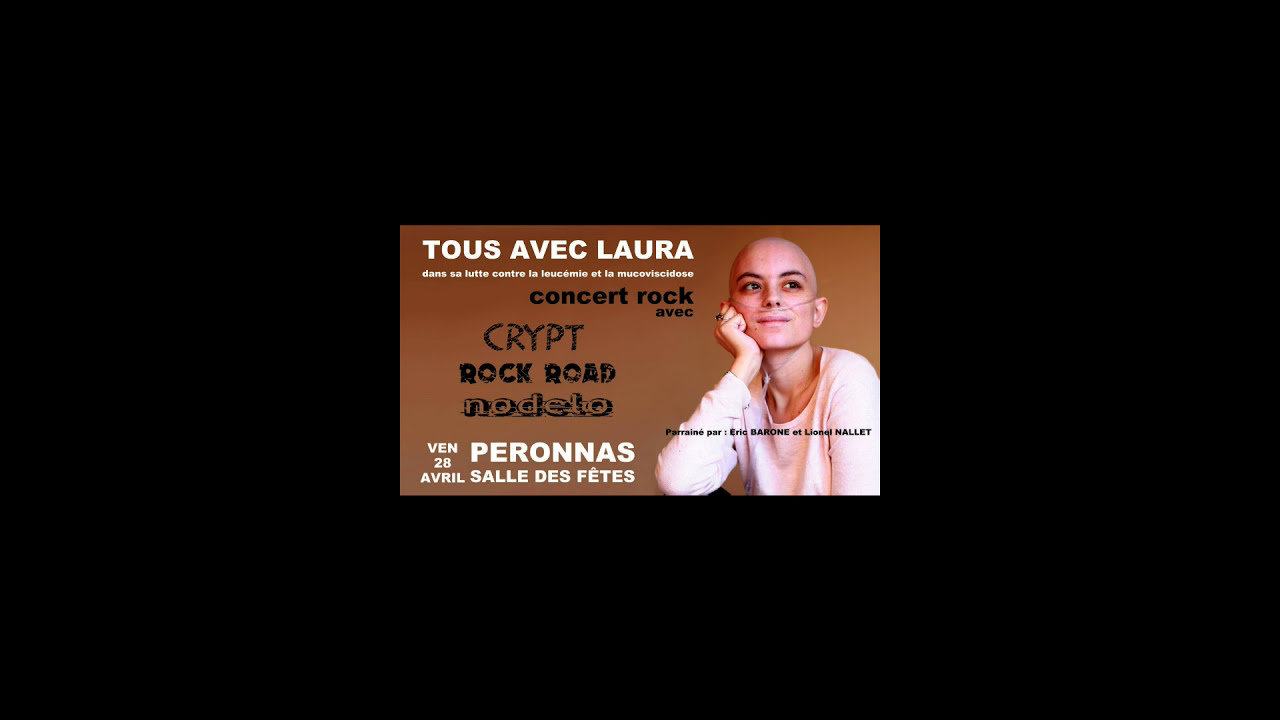The image is a detailed advertisement for a charity event benefitting a woman undergoing a serious illness, likely cancer, as indicated by her baldness and use of a nasal oxygen tube for breathing. The ad features the person, a white female with brown eyes, in the center of a brown gradient background, surrounded by black borders. She is wearing a white long-sleeved shirt, has painted fingernails, and two rings on her left hand, which is supporting her chin as she gazes thoughtfully to the side. Text on the image, largely in a foreign language, includes phrases such as "Tos avek Lara," "Salut contrae le lucemi et la mucoviscovidos," "Concert rock avek Crypt, Rock Road, Nodelo," and "Ven 28 April," indicating a rock concert event scheduled for April 28th. The background of the text is predominantly brown with white and black fonts, giving further emphasis to the charity and concert details.